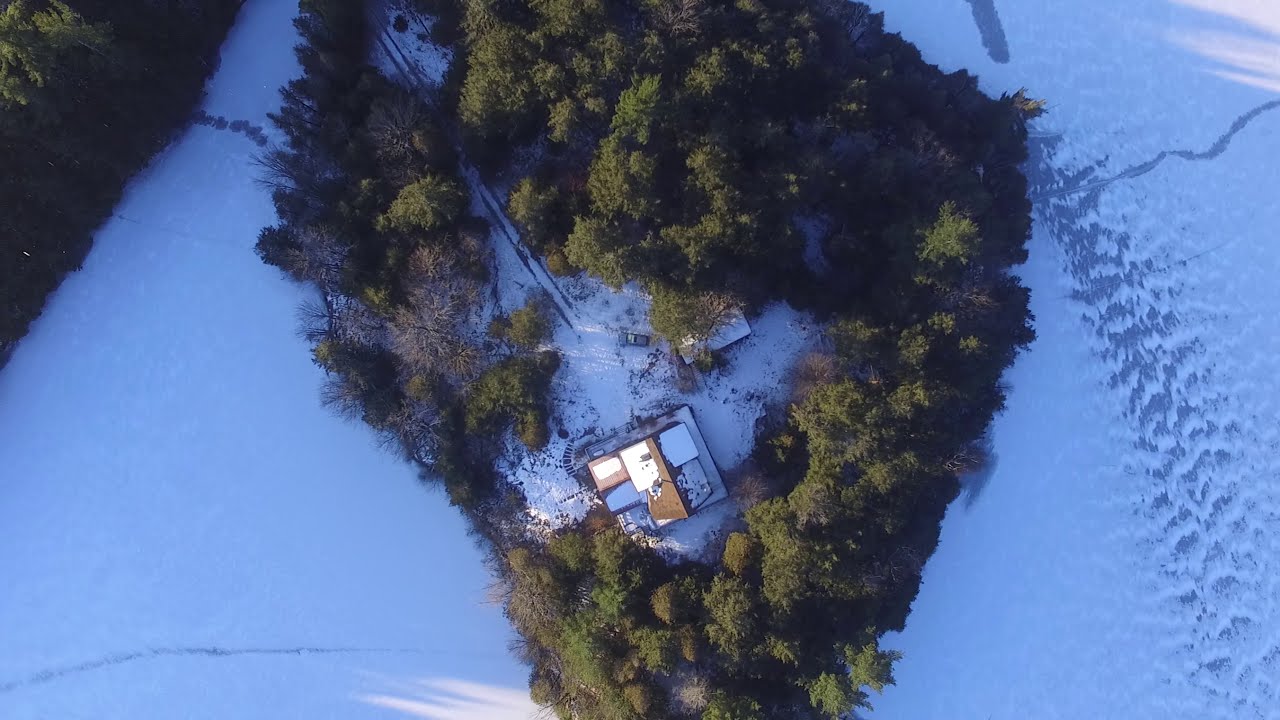This color photograph, captured from a drone in a landscape orientation, showcases a snowy field from an overhead view. At the heart of the image lies a triangular-shaped island of tall, green, bushy trees, almost forming a heart around the contained structures. In the center of this natural enclave, there's a large brown-roofed house, complemented by three additional structures on the left and two on the right. There's also a rectangular structure positioned off to the right-hand side. The entire tree island is surrounded by a fence and enclosed by extensive snow-covered fields. Within the clearing, tire tracks are visible, likely leading to the house or one of the other buildings, with several cars parked out front. The roofs of all the buildings are dusted with snow, accentuating the serene winter landscape captured in this representational realism style photograph.